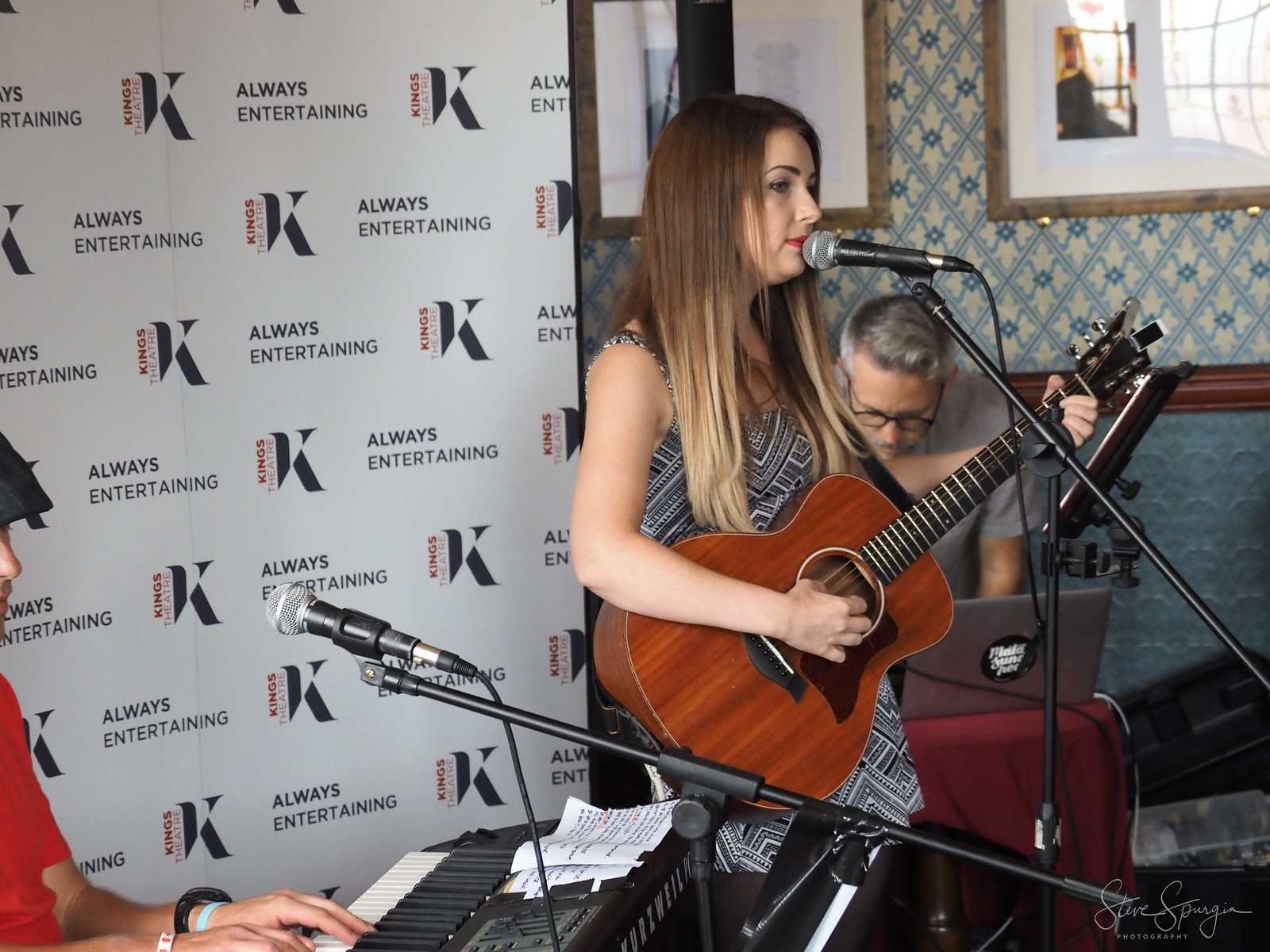A young woman with chestnut brown hair accented by blonde tips stands front and center, gracefully holding an acoustic guitar with gleaming metal strings. Poised before a professional microphone, she exudes confidence and passion. To her left, a man deftly plays an electronic keyboard, accompanied by his own microphone. Behind her, another man intently works on a laptop, placed on a small table draped in a vibrant red tablecloth. The backdrop for this captivating live musical performance is a pristine white screen adorned with logos and the prominent text, "Always Entertaining, King's Theatre."